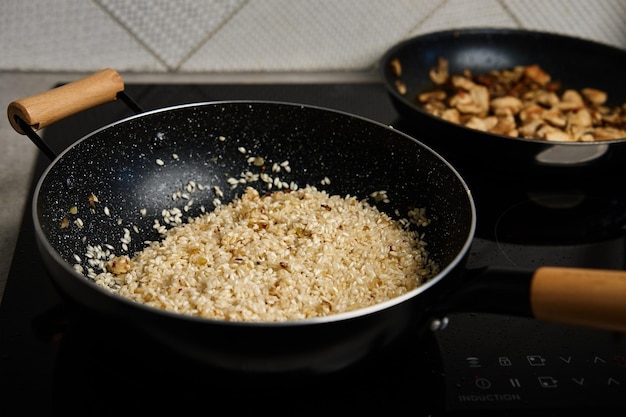The photo is a detailed indoor kitchen scene, highlighting a black glass stovetop with two cooking pans. The background features a tan and white striped pattern running from the top left to the top right, resembling large white checkered squares. The stovetop is modern and sleek, displaying icons at the bottom right where buttons would typically be found.

The pan in the foreground is a black skillet with a silver rim and wooden handles on both sides. Inside, there’s a grain that appears to be a blend of dark brown, light brown, and white, suggesting it could be fried rice or couscous. The grain looks fluffy and seems to be in the process of cooking.

In the upper right-hand corner, the second pan is slightly out of focus and contains light tan, beige, and dark brown ingredients, which seem to be either mushrooms or strips of chicken. This pan is all black, with no visible handles. The stovetop itself is not visibly lit, possibly indicating that the burner is off.